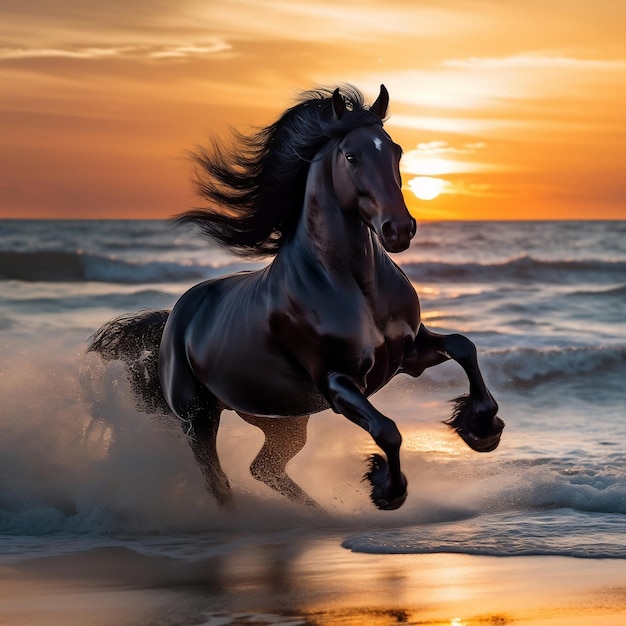This highly detailed and richly colored digital image portrays a black stallion galloping through the water along the shore at sunset. The stallion, with shiny, wet fur and a long, flowing mane and tail, leaps out of the blurred, deep blue ocean, his muscular form glistening under the sun's rays. His front hooves are raised in mid-air, while his rear feet kick up cresting waves, creating a dynamic sense of movement. The sunset sky behind is ablaze with streaks of brass and orange, with wispy clouds framing the bright white and yellow outline of the descending sun. At the bottom of the image, wet sand reflects the radiant colors of the sunset. The main feature of the horse's otherwise smooth black coat is a small white spot between its eyes, adding a touch of distinctiveness to its fierce, untamed elegance.